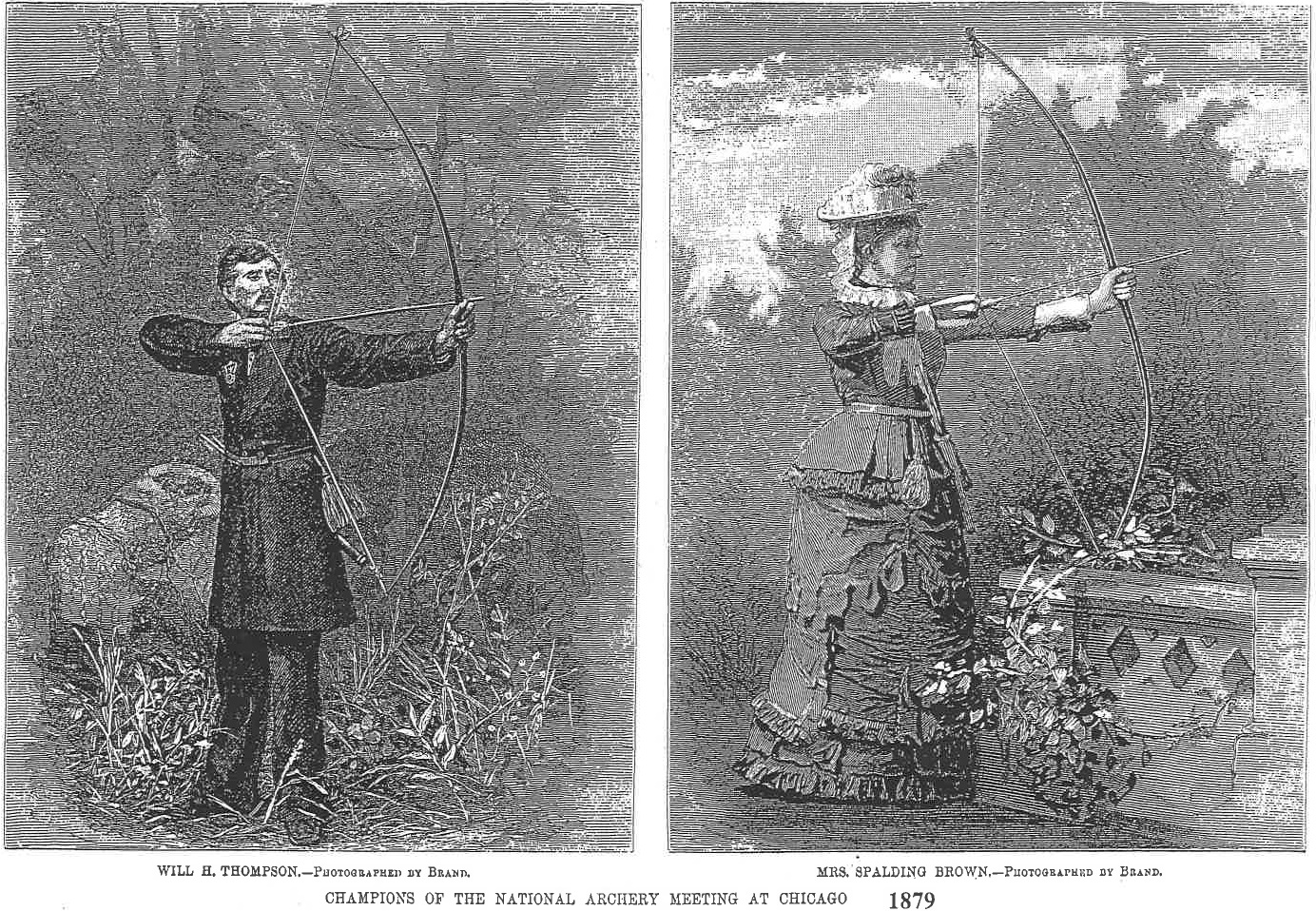The image features two old black and white photographs, seemingly extracted from a book, portraying individuals engaged in archery during an outdoor event. On the left photograph, there's a man named Will H. Thompson, who is depicted wearing a dark-colored coat and pants while holding an old-fashioned wooden bow, drawn back with an arrow ready to shoot. The background includes some trees, bushes, and a potential animal, possibly a dog, near him.

On the right photograph, a woman named Mrs. Spalding Brown can be seen. She is dressed in a long, elegant dress and a hat, similarly holding an old-style bow with an arrow poised to be released. Behind her, trees are visible, and a concrete structure is seen to her right. The bottom of the photographs bears the caption: "Champions of the National Archery Meeting at Chicago, 1879," with detailed credits identifying the photographer, Brand.

This detailed caption highlights the archery preparations of Will H. Thompson and Mrs. Spalding Brown in a natural setting, emphasizing their attire and the historical context of the event.